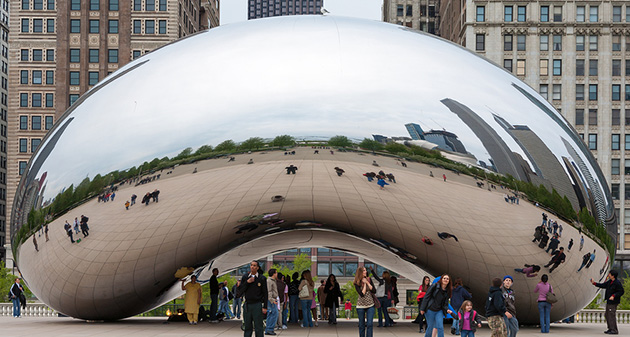This vibrant and professional photograph captures the iconic Cloud Gate sculpture, commonly known as "The Bean," situated in Millennium Park, downtown Chicago. Dominating the foreground, the large, kidney-shaped sculpture features an exquisite silver, mirrored surface that reflects its surroundings, including a bustling crowd of tourists, green-leafed trees, and towering skyscrapers. The reflective nature of the Bean creates a captivating visual play, showcasing slightly distorted images of people walking under and around it. These individuals, diverse in age and ethnicity, are either taking photographs or marveling at the sculpture. Behind the Bean, tall buildings with rectangular windows form a striking urban backdrop, enhancing the image’s depth and context. The photograph, taken during daytime, highlights the vivid, lively atmosphere of a popular tourist spot.